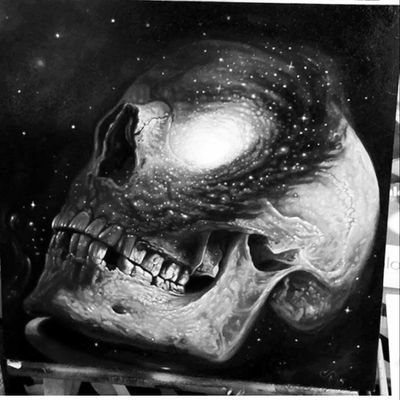This captivating black-and-white image showcases a prominent skeleton featuring a large skull that occupies most of the frame. The skull, rendered in varying shades of gray, displays a distinct missing tooth in the bottom row, creating a noticeable dark gap. The nose area is represented by a flattened, blackened shape, and only the left eye socket is visible, emitting a bright, shiny light amidst the darkness. The surrounding eye area appears like a swirling black hole with white specks, resembling a star-studded sky. The backdrop enhances this celestial effect, portraying a pitch-black night sky dotted with tiny, glimmering stars that elevate the ethereal quality of the scene.